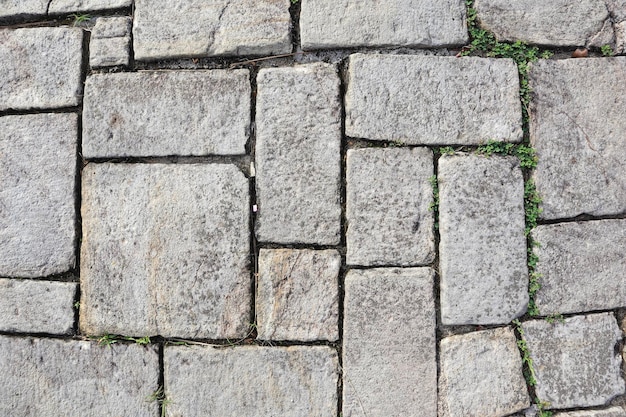This image showcases a detailed view of an outdoor stone pathway or wall, composed of a variety of gray stones meticulously fitted together like pieces of a puzzle. The stones vary widely in size, ranging from perfectly squared pieces to traditional rectangular shapes, with some stones having more irregular forms. They display a white chalky exterior, with some touches of brown mixed in the gray, unified by a consistent stone material. Despite the irregularity in shape and size, the stones are expertly laid with minimal gaps, tightly arranged to create a cohesive surface. Between the grooves where the stones meet, small, green weeds with tiny leaves sprout through, adding a touch of life to the structured scene. The image is likely taken from above, contributing to the perception of the stones forming a patterned walkway, although it retains some ambiguity regarding its exact orientation. The lower right corner features a distinct stone with a sharp end, standing out amidst the otherwise regular geometric arrangement.